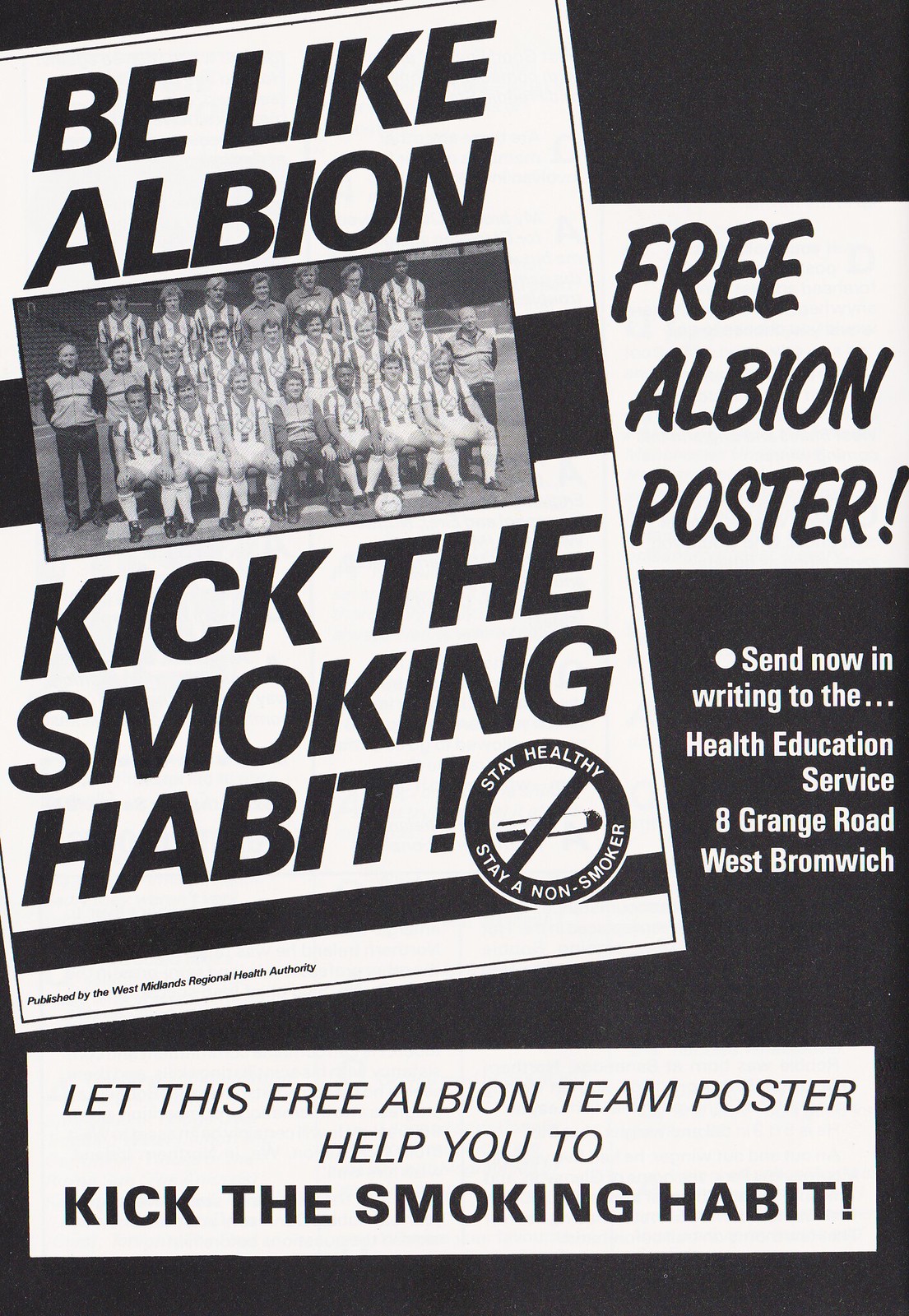This monochrome public service announcement, likely from an old soccer program or magazine, features a promotional poster urging readers to quit smoking. Dominating the left side of the ad is a black and white image of the Albion soccer team posed in three rows. Above the photo, bold, italicized, sans-serif text reads "Be Like Albion," while below it, large, bold letters proclaim, "Kick the Smoking Habit." On the lower right side of the ad, a “Stay healthy, stay a non-smoker” slogan is accompanied by a no-smoking symbol.

To the right of the image, in a white section with black text, readers are informed about how to obtain this free poster: "Send now in writing to the Health Education Service, 8 Grange Road, West Bromwich." Emphasized in script font is a call to action, "Free Albion Poster," which appears once more in italics. The concluding message at the bottom, enclosed in a rectangular box, reiterates the poster's purpose: "Let this free Albion team poster help you kick the smoking habit," underscored by the thicker, bolded text of "Kick the Smoking Habit."